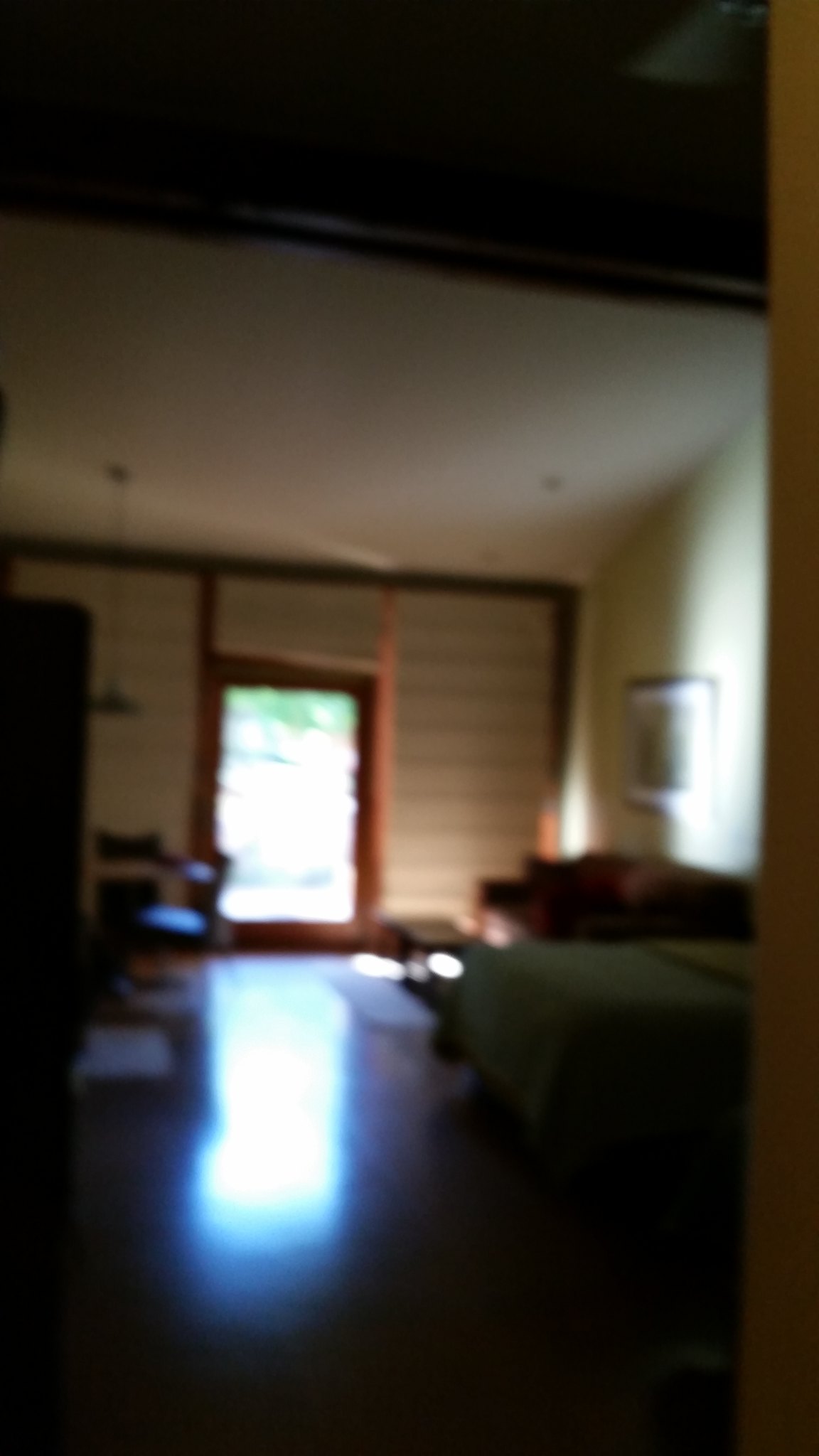The blurry photograph captures the interior of what appears to be a living room within a house or apartment. Dominated by a vaulted ceiling that slopes at a 45-degree angle, the room features several clear elements despite the image's lack of sharpness. The focal point seems to be a large glass door or very large window on the far wall, allowing light to spill in and revealing a glimpse of green vegetation outside. This door or window is flanked by floor-to-ceiling glass panels covered by Roman blinds. 

To the right, there is a bed with a green comforter next to a red couch positioned against a yellow wall, adorned with a framed painting. There's a black swivel office chair and a pendant light fixture hanging from the ceiling. An armchair sits near the large glass door, contributing to the cozy atmosphere. The shiny parquet floor reflects the natural light, enhancing the room's warm and inviting feel. Additionally, a bookshelf is visible, suggesting a blend of function and comfort in the living space.